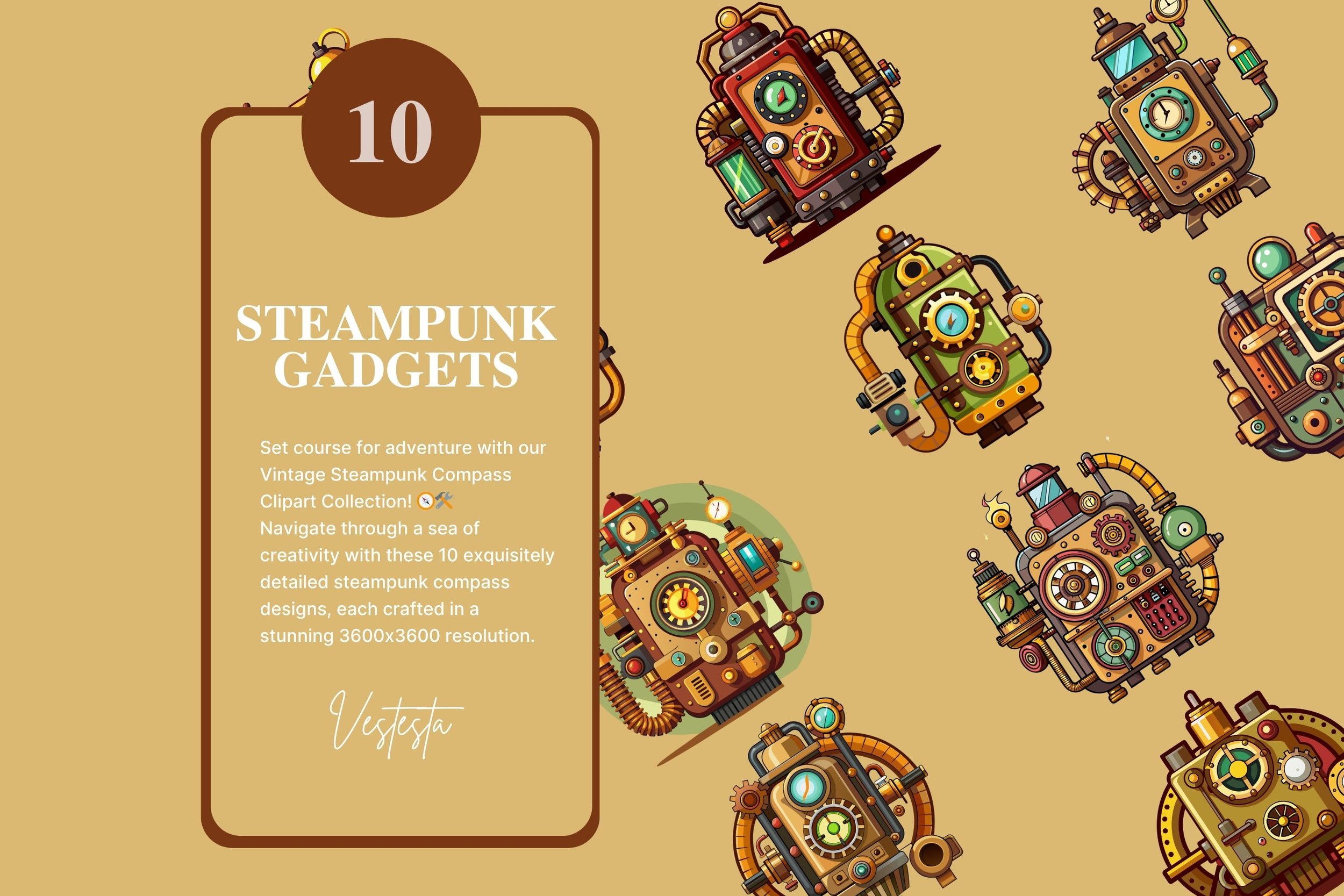This advertisement radiates a Steampunk aesthetic with a dominant yellow background. On the left side, there is a golden-brown rectangle outlined in brown, featuring a prominent circle at the top with the number '10' in white text. Beneath this circle, the headline boldly reads "Steampunk Gadgets." The descriptive text in white invites viewers to "Set course for adventure with our vintage Steampunk Compass Clipper collection. Navigate through a sea of creativity with these 10 exquisitely detailed Steampunk Compass designs, each crafted in a stunning 3600 by 3600 resolution." At the bottom of the text section is the brand's signature, which appears to start with "Vestesta."

On the right side of the advertisement, starting slightly left of the midpoint and extending to the right corner, are various examples of these Steampunk Compass designs. These gadgets incorporate iconic Steampunk elements with dials, tubes, and intricate gears, combining shades of brown, green, yellow, and red to create a vibrant and colorful display. The detailed compass designs exude a vintage, mechanical charm that’s characteristic of the Steampunk genre.